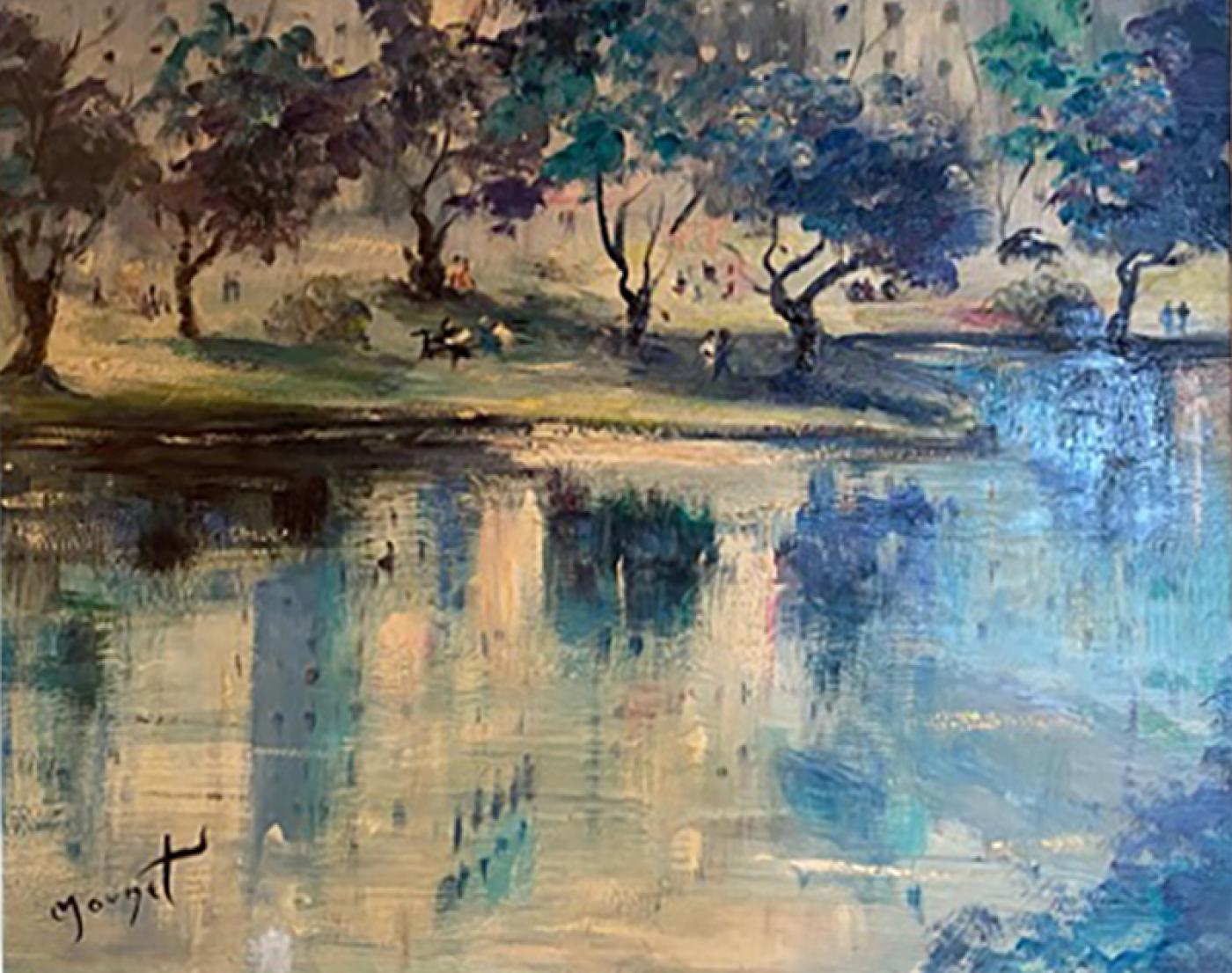This painting, rendered in an expressionist style, features a large body of water, likely a lake or pond, taking up about 70% of the composition. The water is depicted in shades of white and blue, interspersed with reflections of the surrounding landscape. The right side of the water appears to be glowing with an intense blue hue. The shoreline is irregular, jutting in and out, bordered by a grassy area and a variety of trees with dark black trunks. The foliage is a mix of teal, blue, green, and brown tones, creating a rich, textured backdrop.

In the background, numerous people and animals can be seen, though they appear small and distant. Some are possibly accompanied by dogs. The left side of the riverbank provides a shaded area under the trees where people seem to be relaxing and enjoying the scenery. There are also a few birds on the water, identifiable by dark shapes.

The artist's signature is located in the bottom left corner, written in black. Though the signature is somewhat messy and hard to read, it marks the piece with the artist’s personal touch.